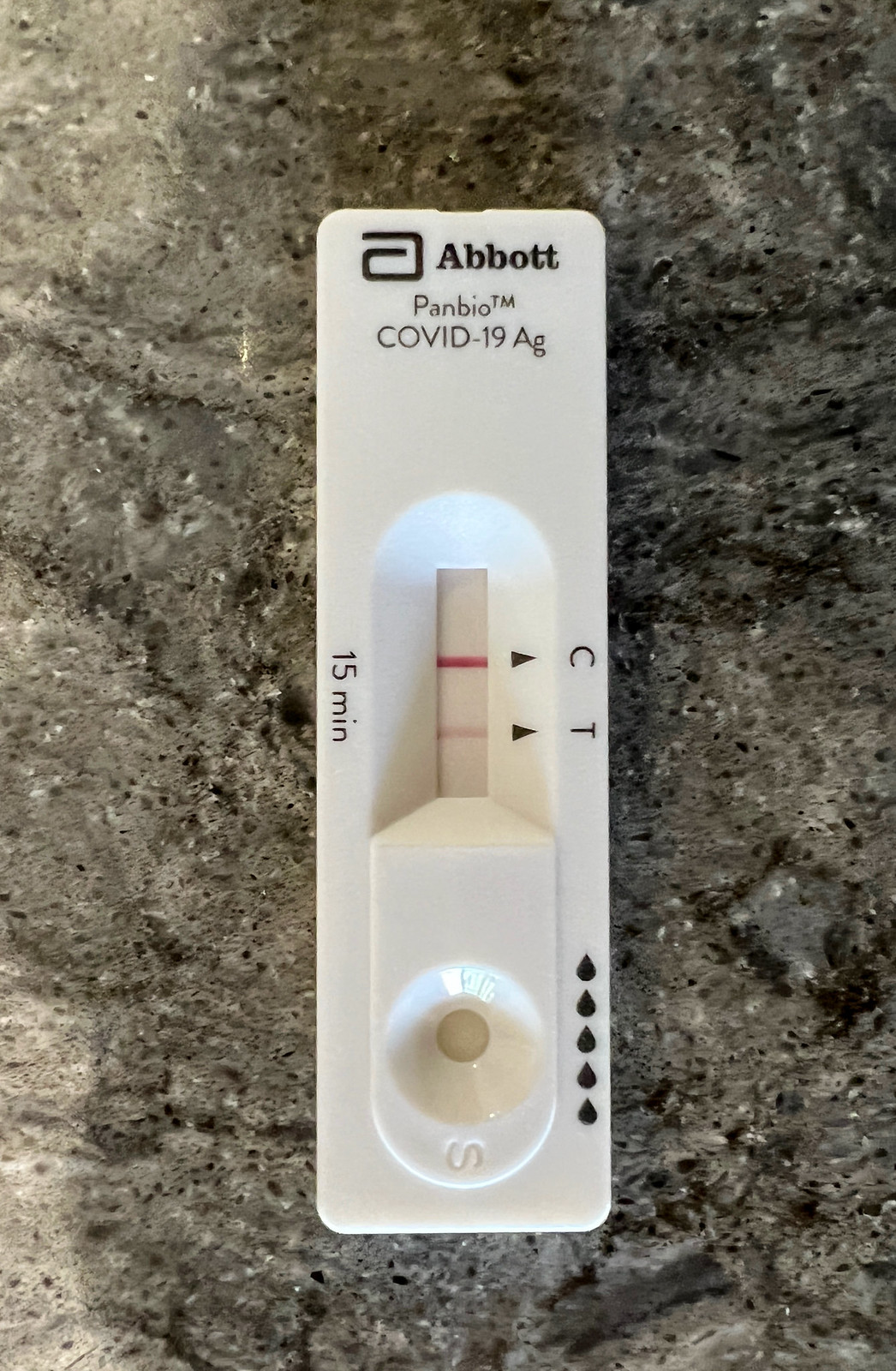This close-up photograph showcases a COVID-19 rapid test placed on a dark speckled countertop, which appears to be made of granite or marble. The test, manufactured by Abbott and branded as Panbio™ COVID-19 Ag, features a long narrow white plastic strip. At the very top of the test, the Abbott logo is clearly visible. Below the logo, the words "COVID-19 Ag" are printed next to the Panbio™ trademark.

The test strip area is prominently displayed, with "15 MIN" written on the left-hand side, indicating the duration of time required for the results. Adjacent to this, a C (Control) and T (Test) are marked with arrows pointing to the corresponding indicator lines. The result of the test is positive, as evidenced by a deep pink line in the control area (C) and a faint pink line in the test area (T).

At the lower end of the test, there is a small well or reservoir intended for the application of the sample drops. Adjacent to this well, five droplet icons are neatly printed in black, guiding the user on the number of drops required. The countertop on which the test is placed is dark grey, interspersed with lighter shades of grey, brown, and white speckles, adding a textured, intricate backdrop to the image.